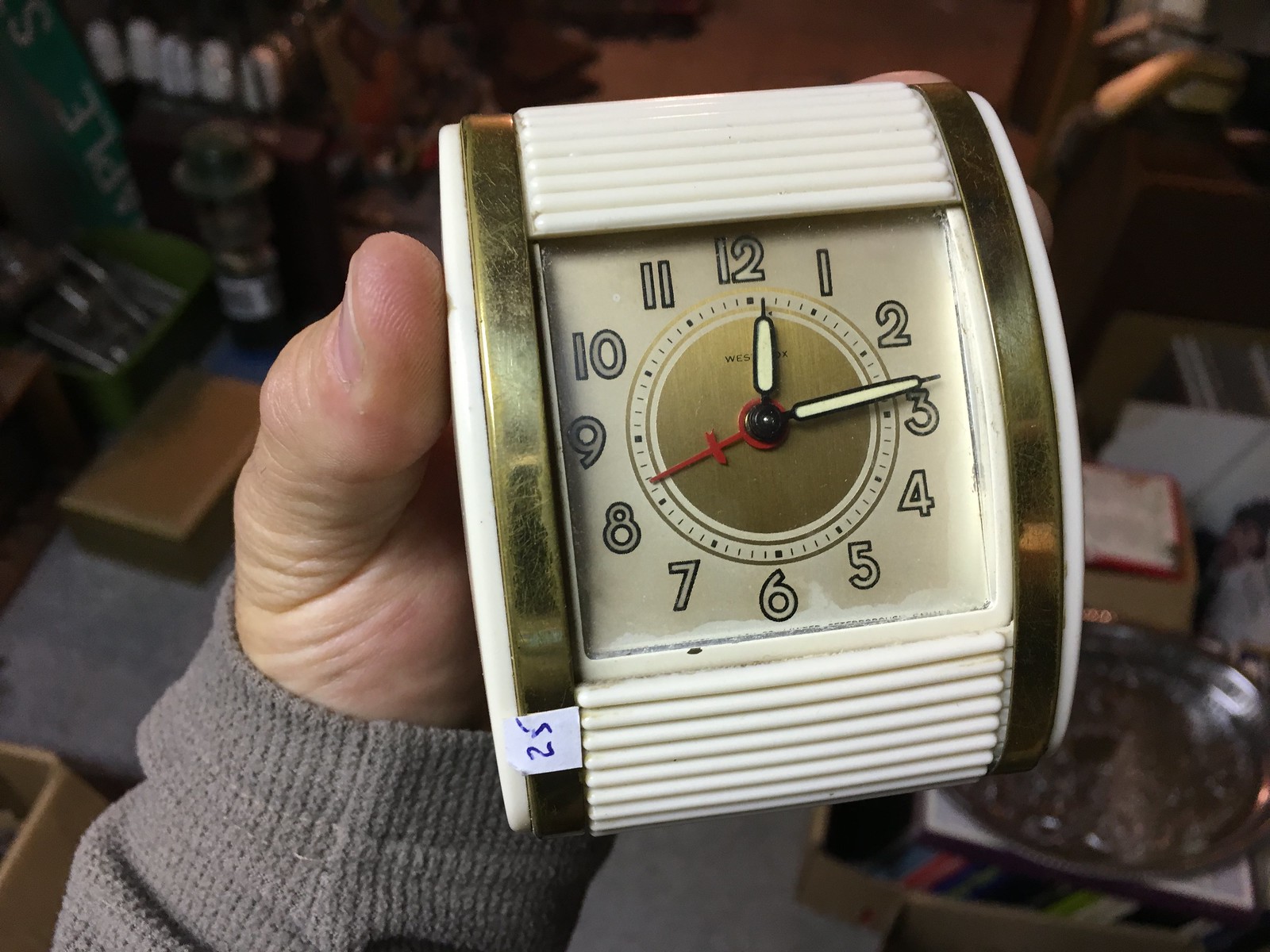This image features a detailed close-up of a clock being held by a person wearing a long-sleeved gray sweatshirt. The clock is characterized by its gold-rimmed body and a predominantly white exterior, with a gold center. The clock face displays the time as approximately 12:14 and 40 seconds. Its design includes white hour and minute hands, a red second hand, and numerals that are white bordered in black. The face of the clock also shows partially legible letters, ‘WES,’ suggesting an incomplete brand name. Notably, the clock's bottom left corner has the number "25" which might indicate its price. The background, slightly out of focus, reveals an assortment of antique items and tools, enhancing the old-world charm of the scene. Overall, the colors featured prominently in the image are gold, white, black, red, and green.